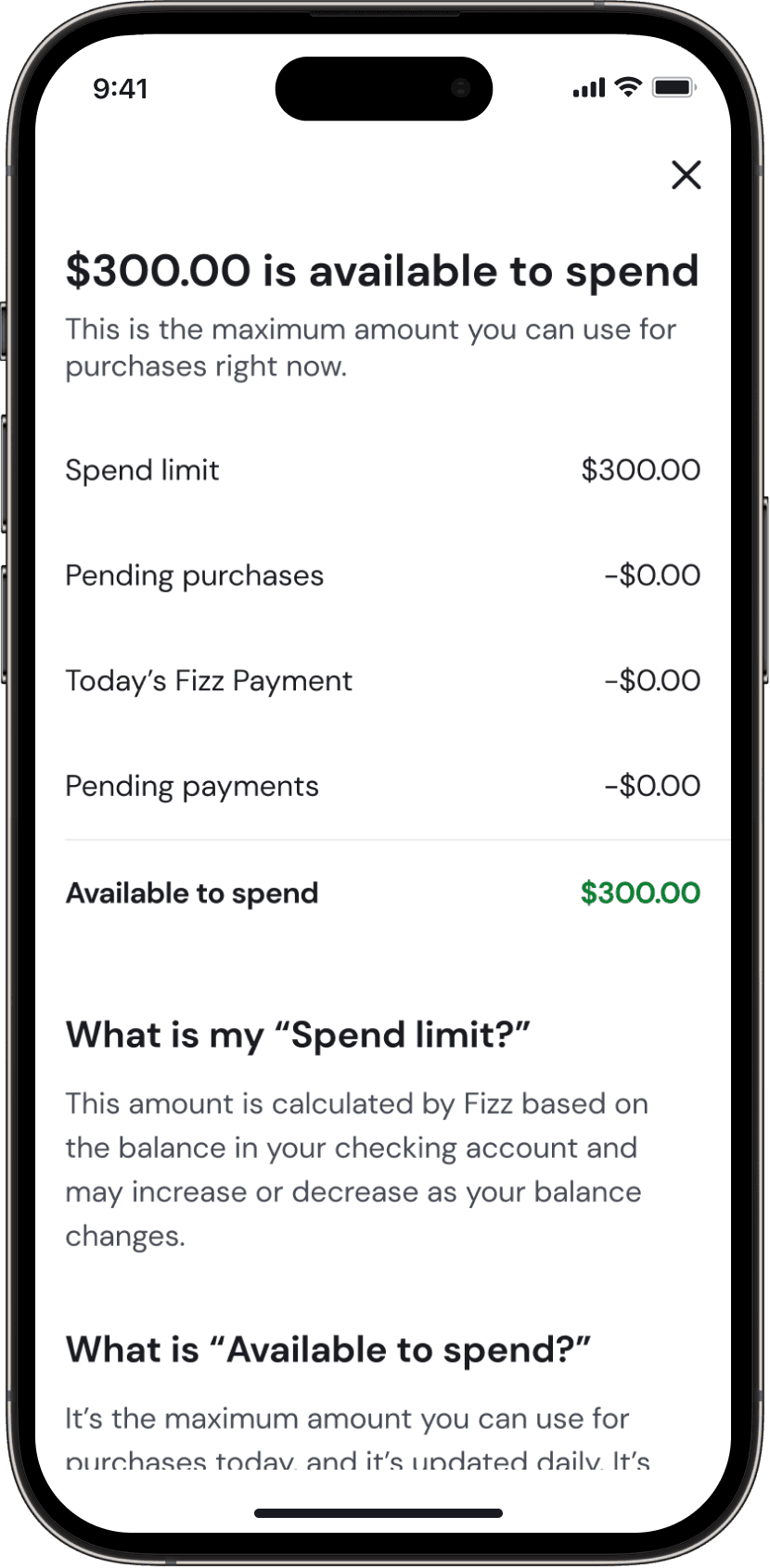Here's the cleaned-up and detailed caption for the image:

---

**Screenshot of a Financial App on a Smartphone**

The smartphone's screen displays a financial app with a black phone outline and a white screen. At the very top left corner, the time is shown as "9:41," next to a small black circular icon. On the top right corner, there are indicators for cellular signal strength, internet connection, and a full battery icon.

Below these indicators is an 'X' icon for closing the screen. Underneath, in bold black letters, the text reads "$300 is available to spend." In smaller gray text below, it explains, "This is the maximum amount you can use for purchases right now."

Further down, the screen displays:
- **Spend Limit:** On the left, "Spend limit" in black, and on the right, "$300" in black.
- **Pending Purchases:** Below, "Pending purchases" with "- $0.00" listed underneath.
- **Today's Fizz Payment:** "Today's fizz payment" showing "$0.00" and "Pending payment" with "- $0.00" listed beneath it.
- **Available to Spend:** In bold black on the left, "Available to spend," and on the right, "$300" in green.

At the bottom of the screen, the app has more information:
- In bold, "What is my spend limit?"
- In gray, "This amount is calculated by Fizz based on the balance in your checking account and may increase or decrease as your balance changes."
- "What is available to spend?" in bold is followed by an explanation in gray: "The maximum amount you can use for purchases today. It is updated daily."

The text appears to continue below the visible area of the screenshot.

---